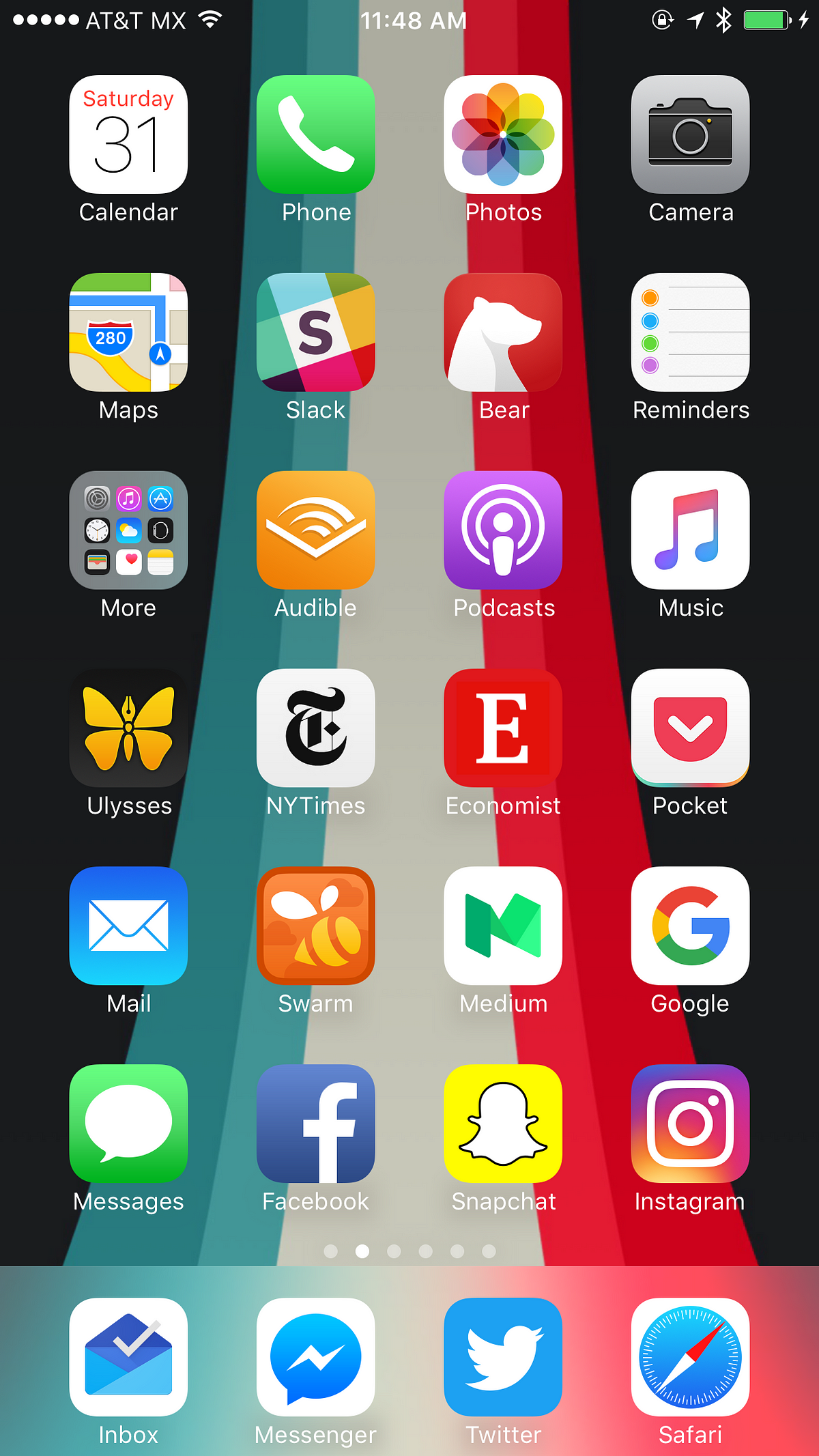The image depicts a smartphone screen with a detailed and organized display. At the top left corner, the signal strength is shown as five solid dots, indicating a strong AT&T MX connection. Adjacent to this, a full Wi-Fi bar is present. The time is displayed as 11:48 AM. On the right side of the header, there are several icons including a lock, location services, Bluetooth, and a nearly full green battery with a charging symbol.

The screen features 24 app icons arranged in a grid, with an additional four apps located on the transparent navigation bar at the bottom. Starting from the top left, the first row includes: Calendar, Phone, Photos, and Camera. The second row comprises: Maps, Slack, Bear, and Reminders. The third row lists: Audible, Podcasts, Music, and Notes. The fourth row has: Ulysses, NY Times, The Economist, and Pocket. The fifth row includes: Mail, Swarm, Medium, and Google. The sixth row presents: Messages, Facebook, Snapchat, and Instagram. 

The four icons on the navigation bar at the bottom are: Inbox, Messenger, Twitter, and Safari. The wallpaper is an abstract design with two blue bars on the left and two blue bars on the right, converging in the middle resembling a rocket pop.

Overall, the screen is neatly arranged with a mixture of productivity tools, social media apps, and essential utilities, all set against a visually appealing background.